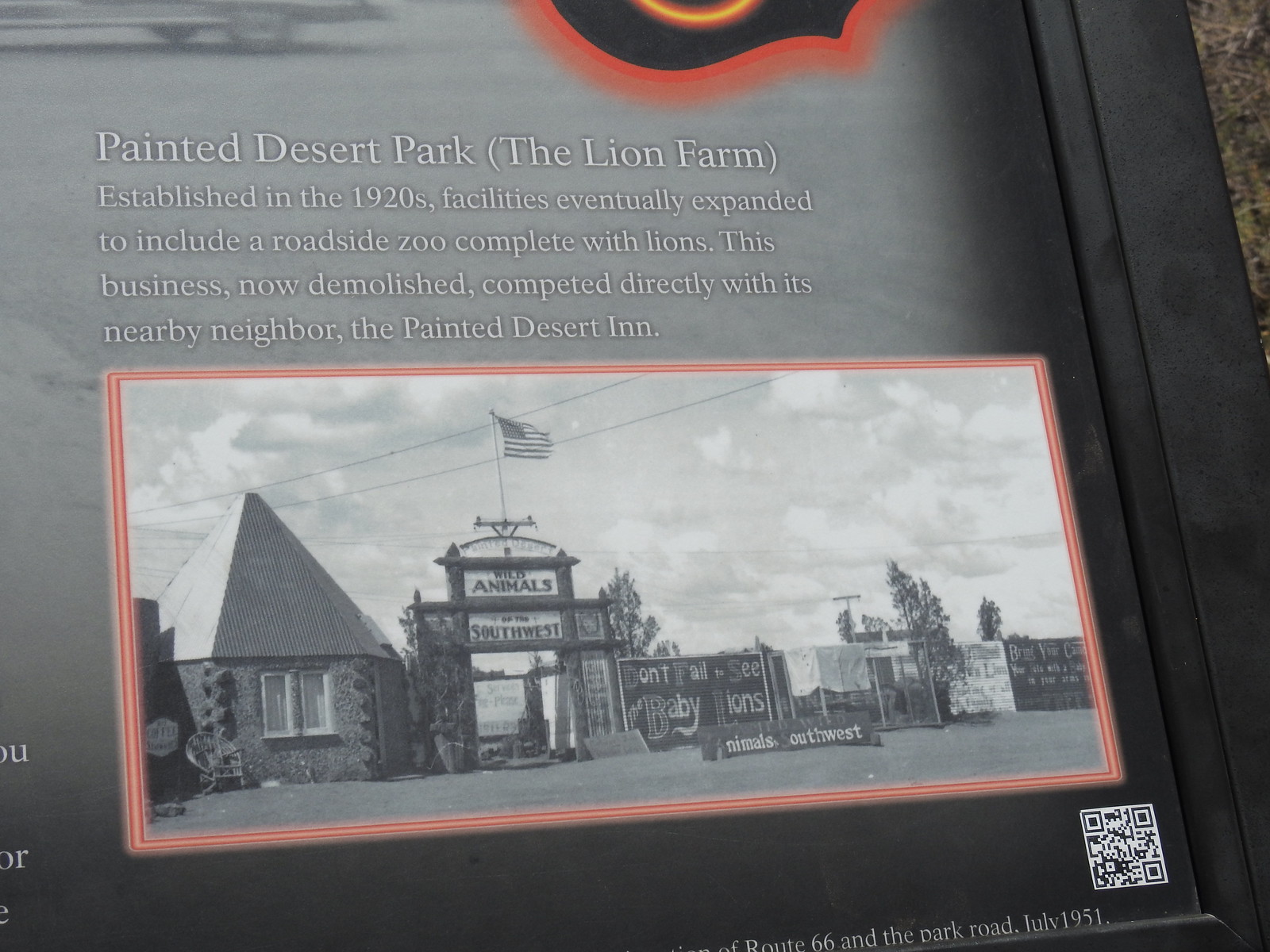The image displays a black plaque set against a background of dirt and grass, featuring a historical account and photograph of the Painted Desert Park, also known as the Lion Farm. Established in the 1920s, the Lion Farm eventually expanded to include a roadside zoo complete with lions, directly competing with the nearby Painted Desert Inn. The photo on the plaque is black and white, displaying a gray, cloudy sky, an American flag on a pole, and electrical cables strewn across the scene. A distinctive cone-shaped concrete building is also visible. Text on the photograph highlights "Animals of the Southwest" and urges visitors, "Don't fail to see the baby lions." A QR code is positioned in the bottom right corner, with a red-bordered logo at the top. Additionally, the plaque notes that the image was taken in July 1951 on Route 66 near the park.